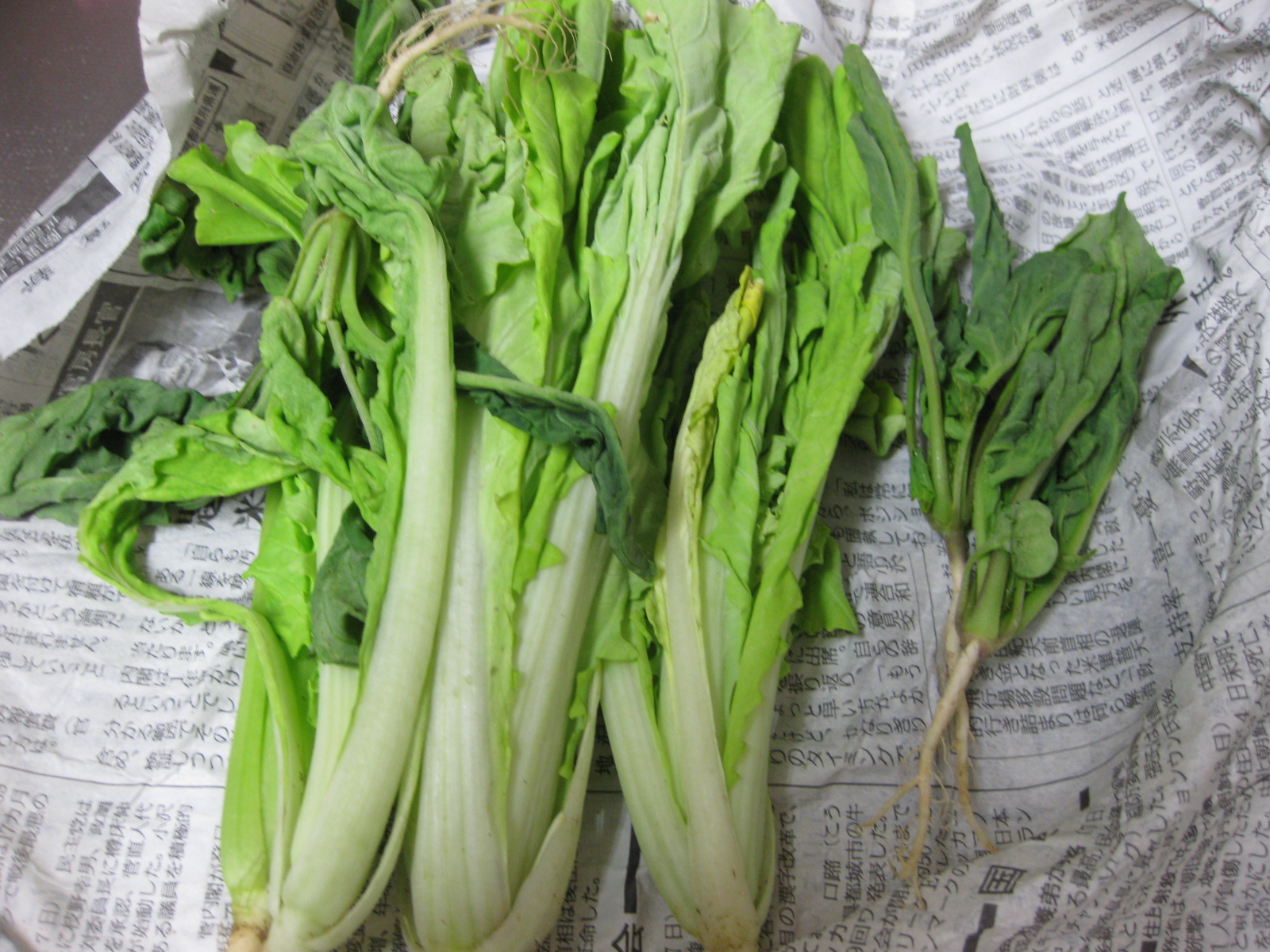The photograph showcases three stalks of wilted celery, characterized by their light green ribs and darker green leaves. These celery stalks, positioned with their cut ends at the bottom of the frame, stretch upwards towards the top of the image. Scattered on the right side are additional wilted leaves that appear to have fallen off. The vegetables are laid out on a black and white Chinese newspaper, indicating they were once wrapped in it. Alongside the celery, there are also some scallions with green tops and white bulbs, further adding to the scene's detail. The overall composition highlights the natural decay and the textured background of the newspaper.